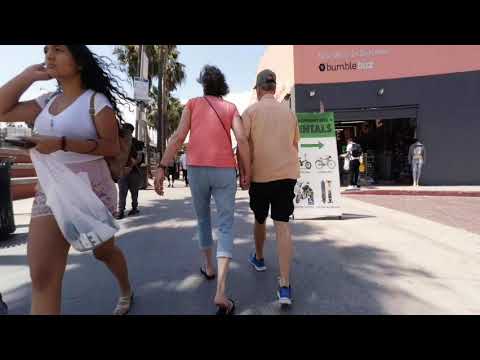In this detailed photograph, three people are walking down a city sidewalk lined with trees and shadows. On the right side, a man, wearing a light orange or tan shirt, black shorts, blue shoes, and a dark gray baseball cap, walks hand-in-hand with a woman. The woman, dressed in a salmon pink short-sleeved shirt and light blue jean capris cut off just above her shins, sports black sandals. In the bottom left corner, a woman with long wavy brown hair, dressed in a white v-neck short-sleeved t-shirt, shorts, and strappy sandals, carries a white bag with black objects inside, possibly on her phone. They pass a storefront named Bumblebuzz on the left, characterized by a tan and pink building facade with a distinctive honeycomb logo. Mannequins in gray and blue outfits stand outside the store, next to a person with a black backpack, white shirt, and black pants. Across the sidewalk, a green sign with "Rentals" and directional signage is visible, likely indicating bike rentals further along the path. The background is adorned with palm trees and their shadows, suggesting a warm, sunny urban environment bustling with pedestrian activity.